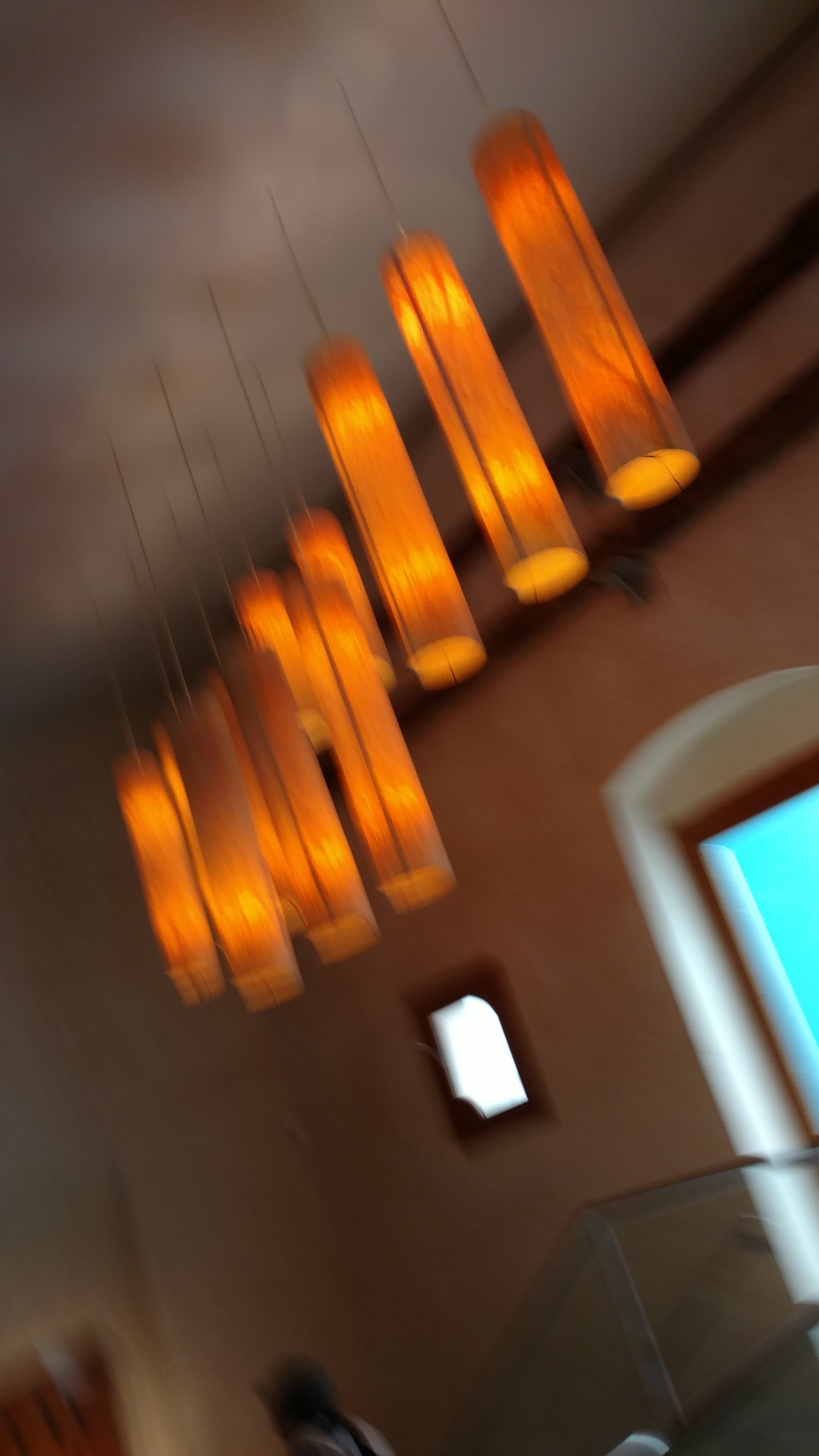In this image, we see a slightly blurry scene that appears to be inside either a home, a restaurant, or possibly a store setting. The image is captured at an angle, adding to the difficulty in discerning specific details. The central focus of the image features striking, long cylinder-shaped lights hanging from the ceiling by thin strings. These lights are a vivid orange hue, and there are approximately eleven of them, with nine being more distinctly noticeable. Towards the background, there are two additional lights partially visible. The room has tan or light brown walls, and in the far right corner, there appears to be a door with a green tint. Above the central lights, there's a small square window adding to the visible architectural elements. Additionally, there is a larger window in the corner with a white outline trim and a light blue color. The combination of orange lighting and these windows is what stands out the most in this somewhat obscure and off-kilter photograph.